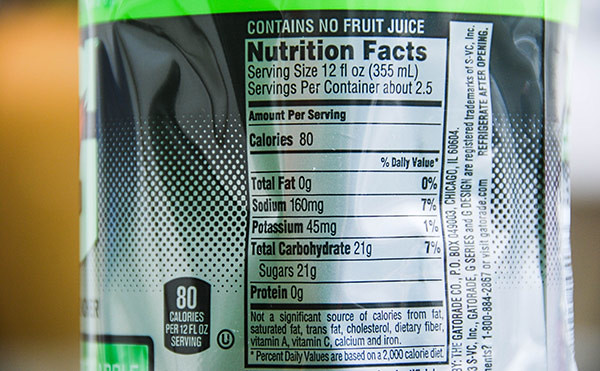The image captures an extremely close-up, high-quality photo of the nutrition label on a Gatorade bottle, suggesting it might even be a screenshot from a commercial. The label, prominently featuring "80 calories per serving," reveals that the bottle contains about 2.5 servings, each serving size being 12 fluid ounces (355 milliliters). The design of the label starts with a green band at the top, followed by a black section with white dots, and transitions to a white background with black dots.

Key nutritional details include: 0g total fat (0% DV), 160mg sodium (7% DV), 45mg potassium (1% DV), 21g total carbohydrates (7% DV), and 21g sugars, with no significant source of calories from fat, saturated fat, trans fat, cholesterol, dietary fiber, vitamin A, vitamin C, calcium, and iron. The label also explicitly states that the drink contains no fruit juice. Additionally, the surrounding blurred background features brown and white tones, with the Gatorade bottle standing out as the main focus. The label includes the address and contact information for Gatorade, confirming the brand of the beverage.